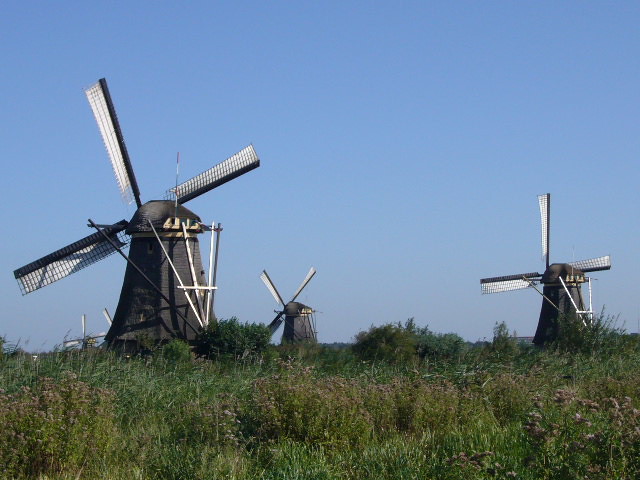This color landscape photograph captures a picturesque scene of windmills in a wild, unkempt countryside, reminiscent of the traditional Dutch windmills used for electricity generation. The foreground features a variety of wild grasses and weeds, with some blades of dark green grass standing at least a foot high. Interspersed among the grass are wildflowers or weeds with brown-tinged tops, complemented by slightly taller bushes in the background.

Prominently, three windmills are clearly visible in the mid-ground: one on the left closer to the camera, one on the right, and another just off-center to the left. In the far left background, two additional windmills are barely discernible, with just their blades peeking out. These windmills, made from concrete, have a bell-shaped base that tapers towards the top. Their fan blades are attached to black arms and are white in color. The windmills also feature additional black and white supports.

The setting is under a clear, sunny sky, which transitions from a darker blue on the left to a lighter hue on the right and near the horizon, creating a striking contrast with the rustic landscape and the mechanical elegance of the windmills.